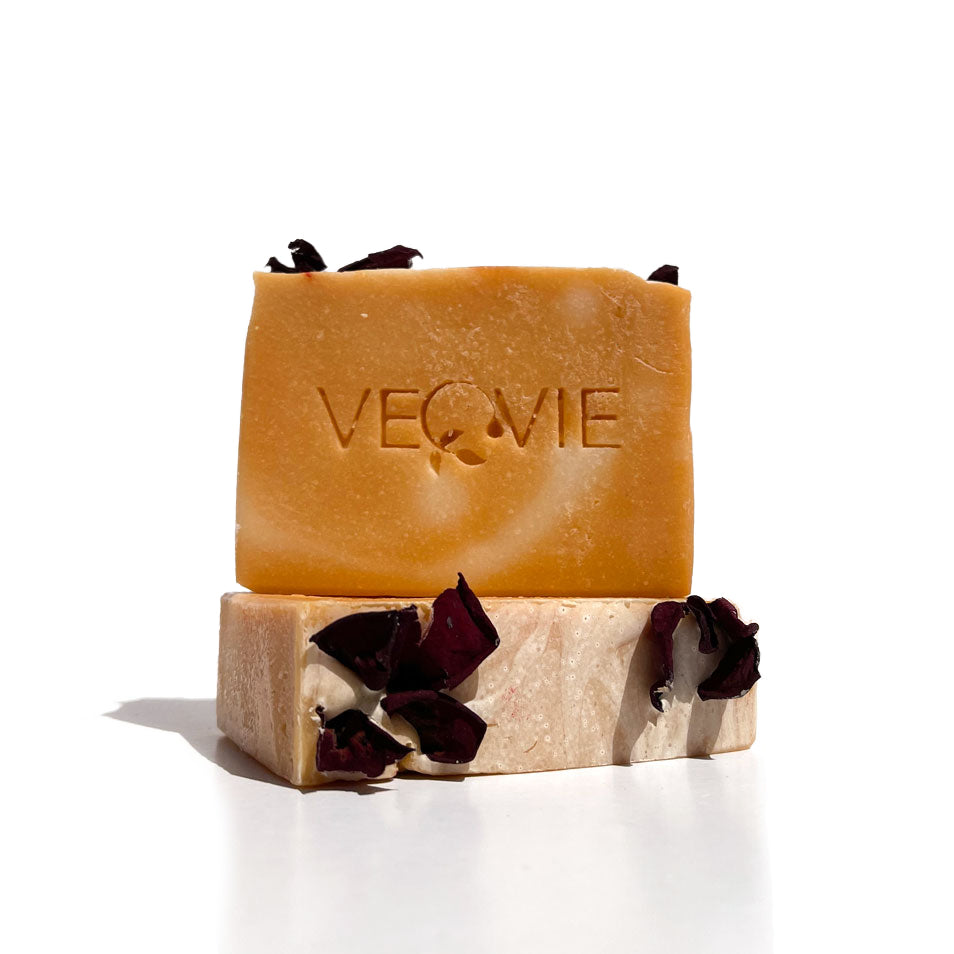This image features two handmade soap bars set against a white background. The bottom bar, which serves as a pedestal for the top one, is a marbled brownish color with a handcrafted, irregular shape. It appears to have dark red or maroon flower petals embedded within it. Resting on this bar is an orangey beige soap, adorned with white streaks and an engraved inscription that seems to read "V.E.C." or "V.I.E." This bar is more vibrant and slightly bolder in color compared to the bottom one. The engraving is surrounded by an intricate leaf pattern, and similar flower petals are also visible on this bar, with two on the top left and one on the top right. The overall arrangement and details suggest an artisanal quality to the soaps, emphasizing their handcrafted nature.